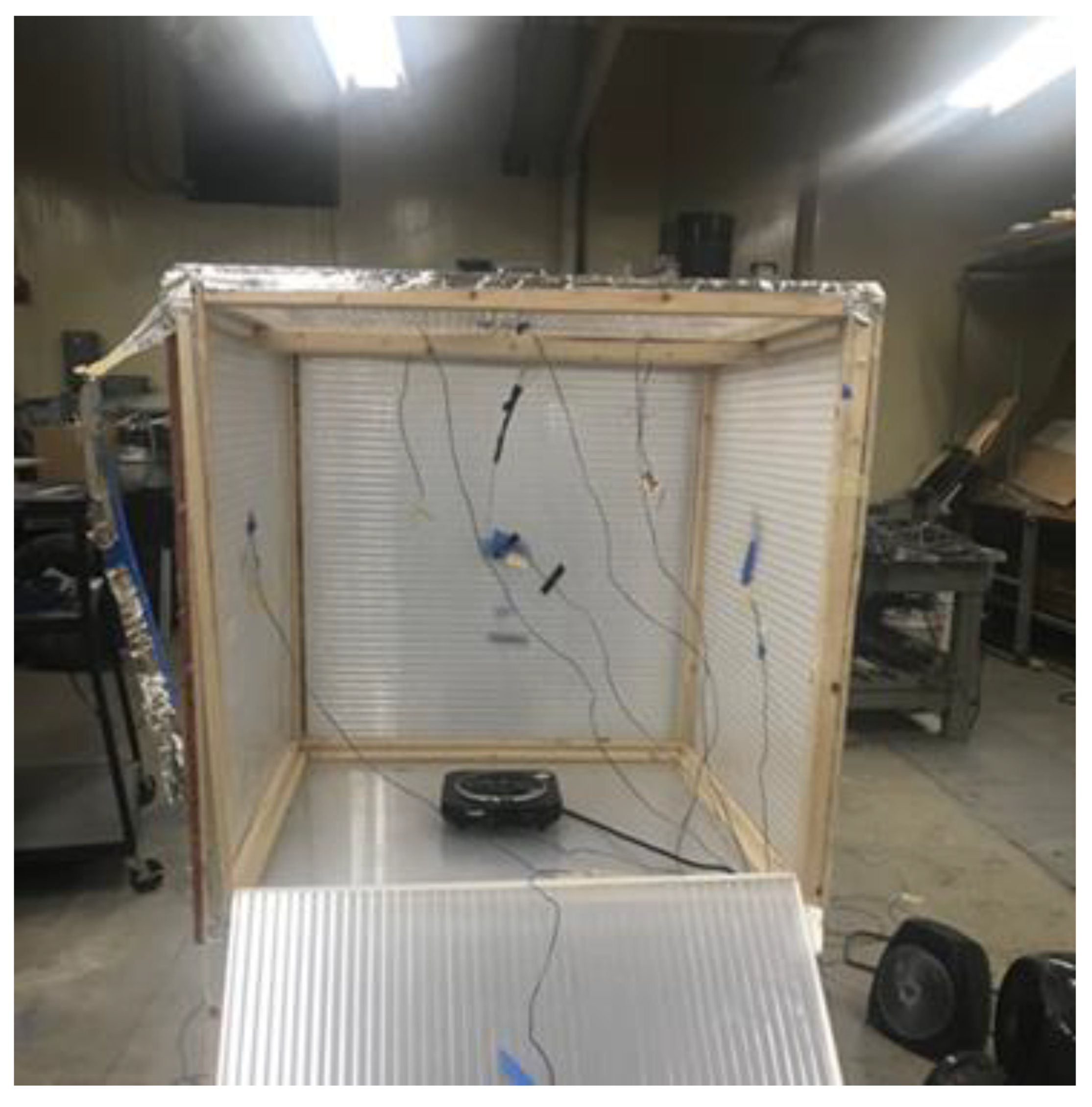In an industrial workshop illuminated by fluorescent lights, the photograph captures a meticulously constructed box-like device dominating the center of the image. This cube-shaped structure features a wooden frame with translucent plastic panels on all sides, designed to allow a soft, muted light to emanate when illuminated. The front panel of the device is hinged and open, revealing its intricate interior. Suspended inside the cube are numerous black wires converging at a small, black, rounded object in the center, resembling an echo dot or power base. Additionally, a tiny light source is visible amidst the wires. The background fades into gray, revealing glimpses of industrial-style work tables and assorted construction equipment, suggesting a space devoted to creative experimentation and repair work.